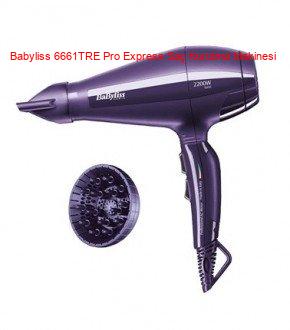This is a color product photograph of a purple Babyliss 6661 TRE Pro Express hairdryer displayed in profile against a white background. The hairdryer has a sophisticated, reflective finish and is shaped somewhat like a futuristic ray gun, with the back end being wider and narrowing down towards the pointed nozzle on the front. The text "Babyliss 6661 TRE Pro Express" is overlaid in orange lettering on the body of the hairdryer, although parts of it are blurry and unreadable. Additionally, "Babyliss" is written in white script on the side, along with a note indicating it is 2200 watts. The handle is equipped with two switches, and the cord extends from the base, protected by a rubber bushing to prevent fraying. The image also shows a separate attachment, a circular diffuser with multiple air outlets, positioned in the lower left corner. This diffuser is designed to spread out the airflow, softening and redirecting it. The entire composition is clear, providing detailed visual information about the product features.